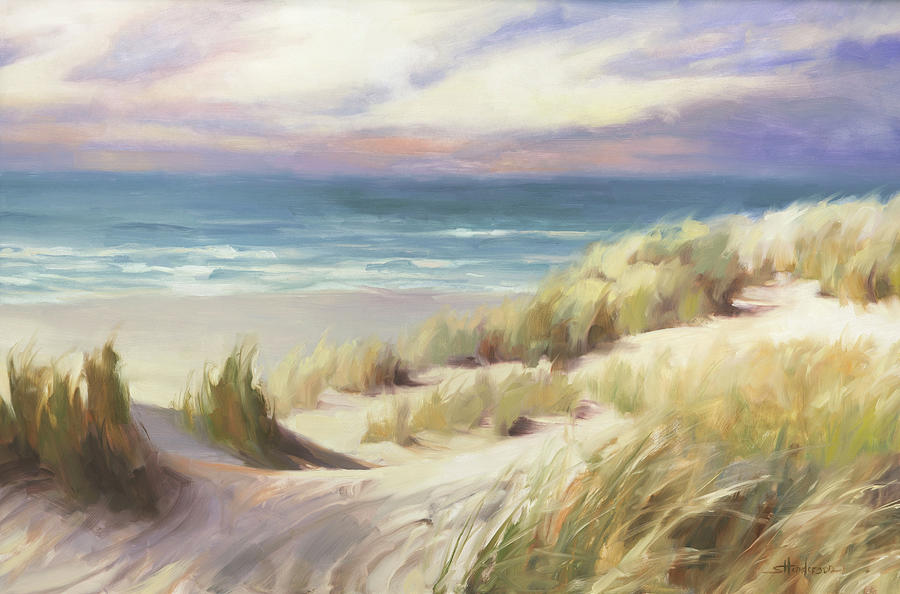This horizontally aligned rectangular painting vividly portrays a beach scene under a dynamic sky. The upper portion is a striking sky with feathery white clouds blending into a blue background, accompanied by sections tinged with brownish-pink, orange, and purple hues, suggesting an early morning or late afternoon ambiance. Beneath this atmospheric sky, the middle section of the painting features a restless ocean, primarily depicted in blue with hints of gray. The waves, capped with white tips, crash energetically against the shore.

Descending from the horizon to the foreground, the shoreline reveals a small patch of beige-colored sand towards the left, providing a stark contrast to the choppy waters. The beach itself transitions into a sandy dune, a hill covered with grass and vegetation, predominantly green and brown, which bends and sways as if in a strong wind. At the base of this dune, in the lower left-hand corner, there are subtle indentations resembling footprints or wind-formed ripples in the tan sand. The scene is completed with brushstrokes that simulate the texture and movement of grass tussocks caught in the breeze, emphasizing the natural, windswept beauty of this coastal landscape.